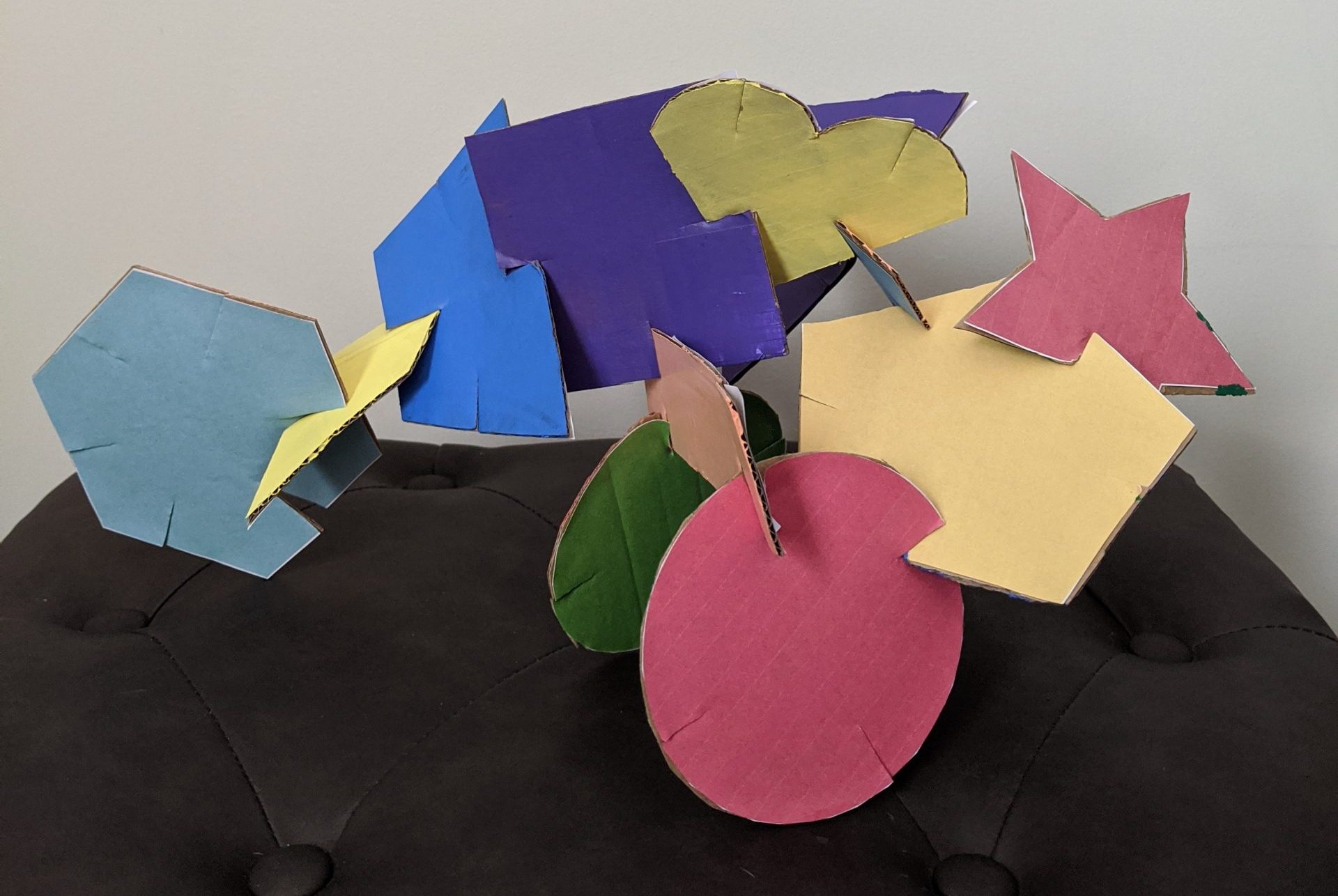This photograph depicts a vibrant and colorful 3D sculpture made from various cardboard shapes, each covered in construction paper in different hues. The shapes, which include hexagons, circles, stars, hearts, squares, and a trapezoid, are connected through notches cut into them, creating an intricate and jumbled arrangement. The cardboard itself appears to have been messily cut, with jagged edges adding to the handmade quality of the art piece. The piece is displayed on a quilted black ottoman, possibly made of microfiber, in front of a white wall. Key connections in the sculpture include a pale blue hexagon attached to a yellow shape, which transitions to a royal blue trapezoid, a navy blue square, and finally to a yellow heart. There are additional connections: a red circle joined to a green circle via an orange rectangle, a yellow pentagon linked to a red star, and another blue square bridging elements. Different colors such as rose pink, dark blue, and green, add to the lively and patchwork aesthetic of the piece.